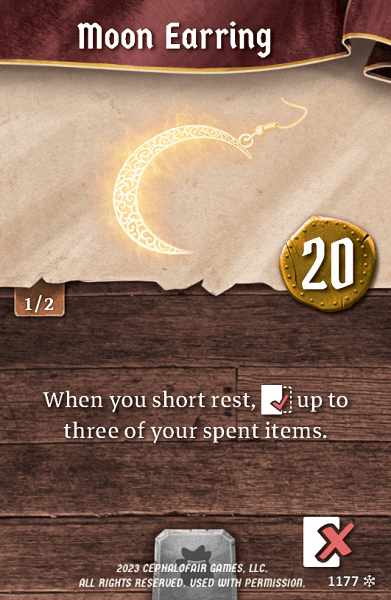The image is a vertically-oriented, rectangular photo featuring a mix of natural textures and labeled elements. The bottom half showcases a horizontal arrangement of wooden beams, resembling a rustic table surface. Situated on this surface is white text stating, "when you short rest," followed by a checkmark symbol and the phrase, "up to three of your spent items."

Above the wooden table, the background transitions to a tan cloth-like material, providing a softer contrast. Centered on this backdrop is a luminous crescent moon earring, highlighted by its sparkling details and a small hoop at the top, giving it the appearance of a dangly charm.

At the very top of the image, the lower edge of a red and gold curtain descends, bearing the label "moon earring" in white text. Positioned between the wooden bottom and the tan upper part, slightly towards the right, is a rough-textured, irregularly-shaped gold coin inscribed with the number "20" in white.

In the bottom right corner, a small white rectangle adorned with a red 'X' is slightly offset towards the right. Additional text is located at the bottom of the image, though it's not detailed in this description.